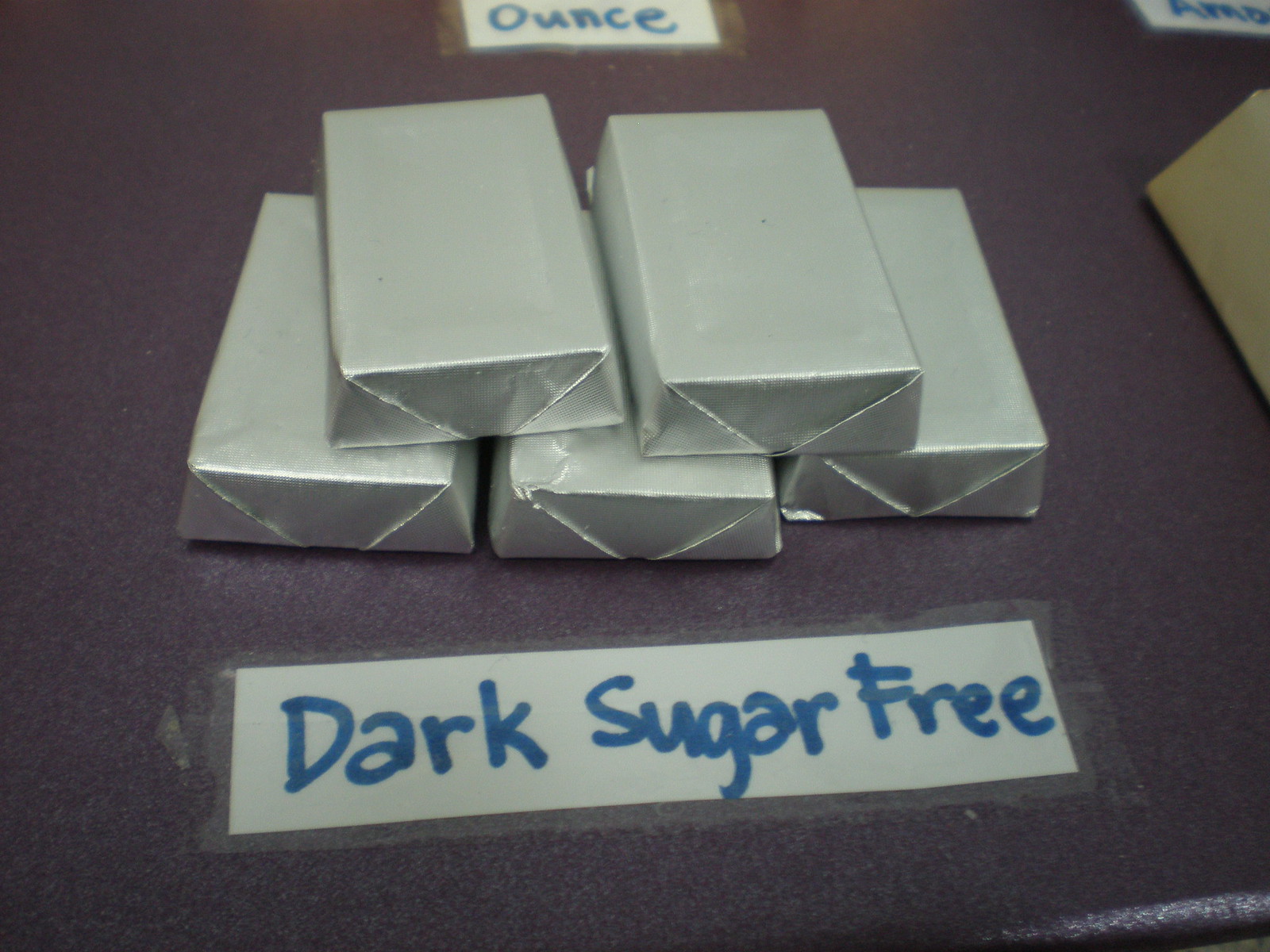This photograph captures five rectangular objects that look like chocolate bars, wrapped in silver aluminum foil, arranged in a stacked formation with three on the bottom and two on top. They are placed on a dark surface, which appears to be a dark brown or black table, possibly a fold-out table. Below the bars, a white label with blue lettering reads "dark sugar-free," suggesting that these might be dark sugar-free chocolate bars, although it’s not explicitly stated. Above the bars, another white label with blue lettering partially shows the word "ounce," although it’s cut off, making it hard to determine the exact meaning or how it relates to the items. Additionally, some more chocolate bars are hinted at the right edge of the image but are partially cut off in the photograph. The overall scene is taped down with translucent tape, giving the image a real, homemade feel.